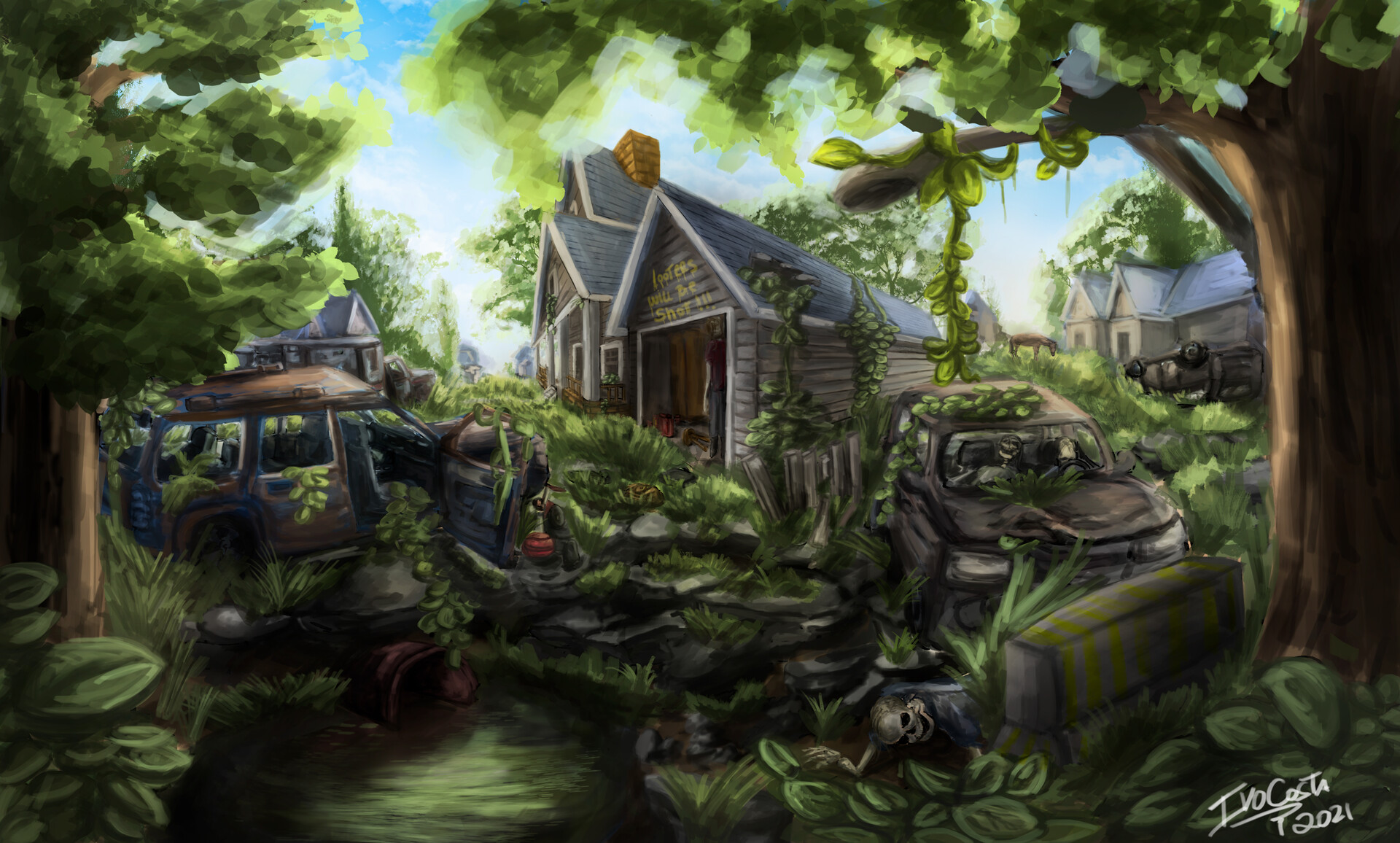This painting by Ivo Costa, signed '2021' in the bottom right corner, depicts a detailed rural landscape scene centered around an old, wooden cottage with gray walls and a triangular blue roof featuring a yellow chimney. To the left of the house stands a large tree with green, fluffy leaves and a brown trunk, casting some of its branches over the cottage. The ground is mostly covered in vibrant green grass and various shrubbery. Scattered vehicles lie in ruins around the area: a brownish, rusted car is positioned to the right of the house by another tree, and other dilapidated vehicles are visible further in the background among more overgrown bushes. A small pond lies at the bottom side of the image, where a human skeleton can be seen on the ground nearby. In the background, more similarly styled houses with gray and tin roofs are visible, partly obscured by trees. The blue sky above is dotted with white clouds, adding to the serene yet eerily abandoned atmosphere of the scene. The garage door of the cottage ominously displays the words "looters will be shot" painted in yellow, hinting at a past conflict or abandonment.